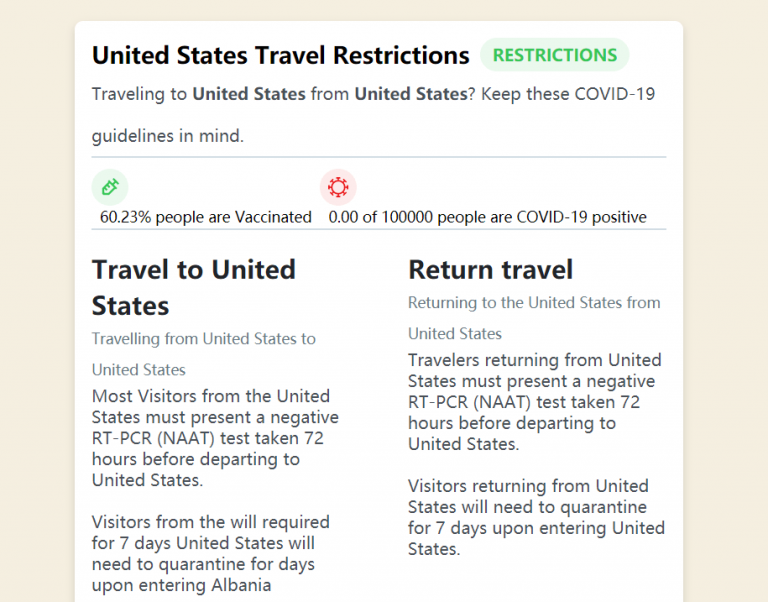The image being described features a tan background with a prominent white document-like section in the center. The document has a header in bold black font that reads "United States Travel Restrictions." To the top right, the word "Restrictions" is written in green fine print. Below the header, the text states "Traveling to United States," and "from United States," both instances of "United States" are in bold. 

Below these lines, there are two icons: on the left, a green icon possibly representing a vaccination shot, and in the center, a red icon resembling a sun, likely the COVID-19 logo. Underneath these icons, a statistic is displayed indicating that 60.23% of people are vaccinated and that there are 0 COVID-19 positive cases per 100,000 people.

In the left section of the document, in dark font, it reads "Travel to United States," followed by a text block detailing steps for traveling from the United States to the United States. To the right, in black font, it states "Return Travel," and in gray font below, "Returning to United States from the United States." Two paragraphs explain the return travel process.